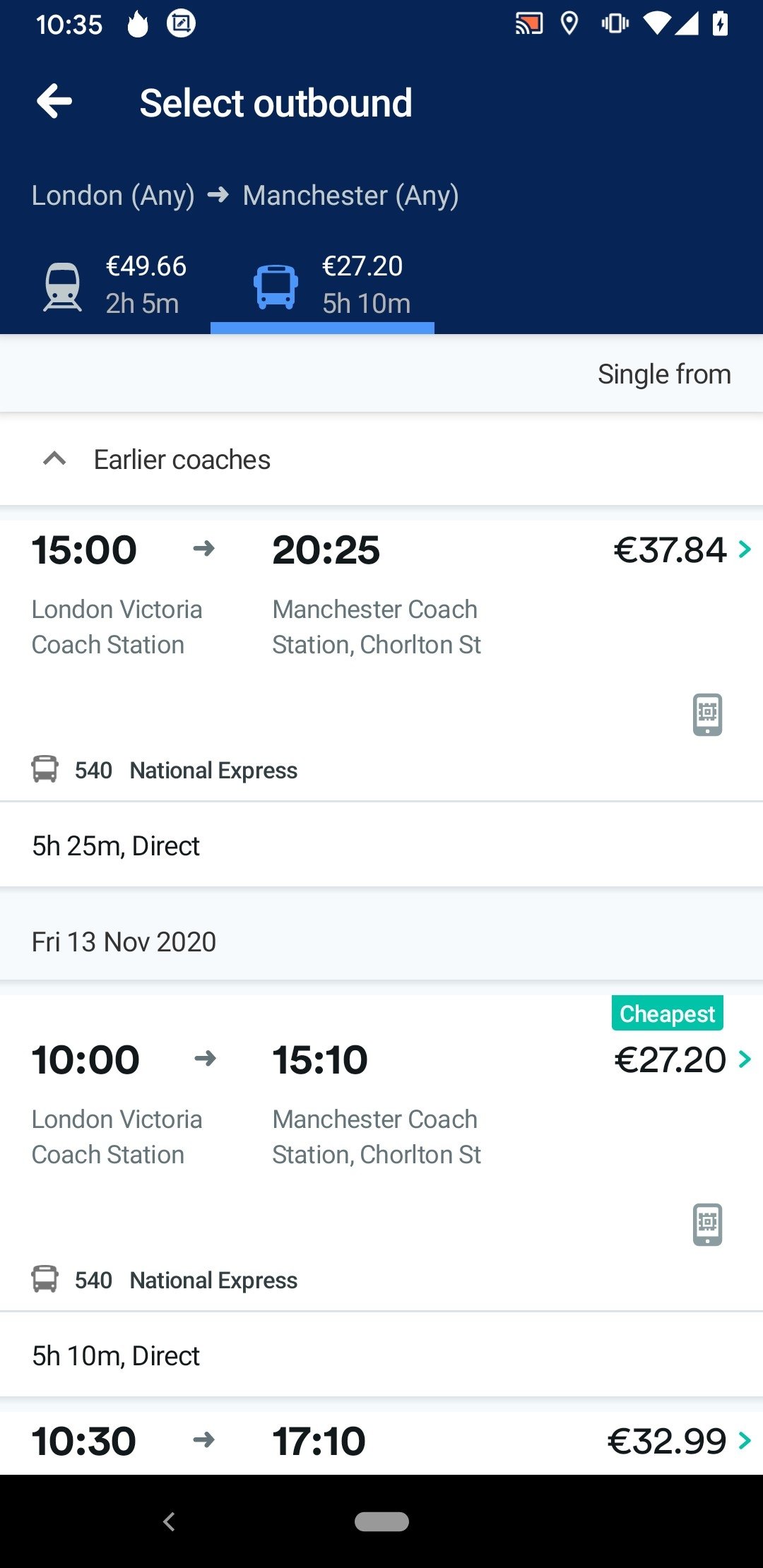The image displays a screenshot of a mobile device, recognizable by the status indicators at the top, which include the time (10:35), Wi-Fi signal strength, and battery charge level. A prominent blue navigation bar at the screen's top shows a back button and the text "Select outbound" in white. Below this, it details travel options from "London, any" to "Manchester, any" with icons for a train and a bus.

Specifically, the train journey is marked as 2 hours and 5 minutes with options priced at $49.66 and $27.20. The bus journey takes significantly longer at 5 hours and 10 minutes. The main content area beneath the blue bar is white and begins with a heading for "single from," followed by an "earlier choices" section marked by an upward-pointing arrow. Time slots and varying prices are listed sequentially.

Detailed information includes a 5-hour and 25-minute direct bus journey via National Express on Friday, 13 November 2020, priced at $27.20 for a trip from 10:15 to 15:40. Another similar direct bus option, running from 10:30 to 17:10, is priced at $32.99. The bottom of the screen ends with a black bar, highlighting the dominant selection of bus travel. This meticulously outlines various times, durations, and costs associated with traveling from London to Manchester by bus.